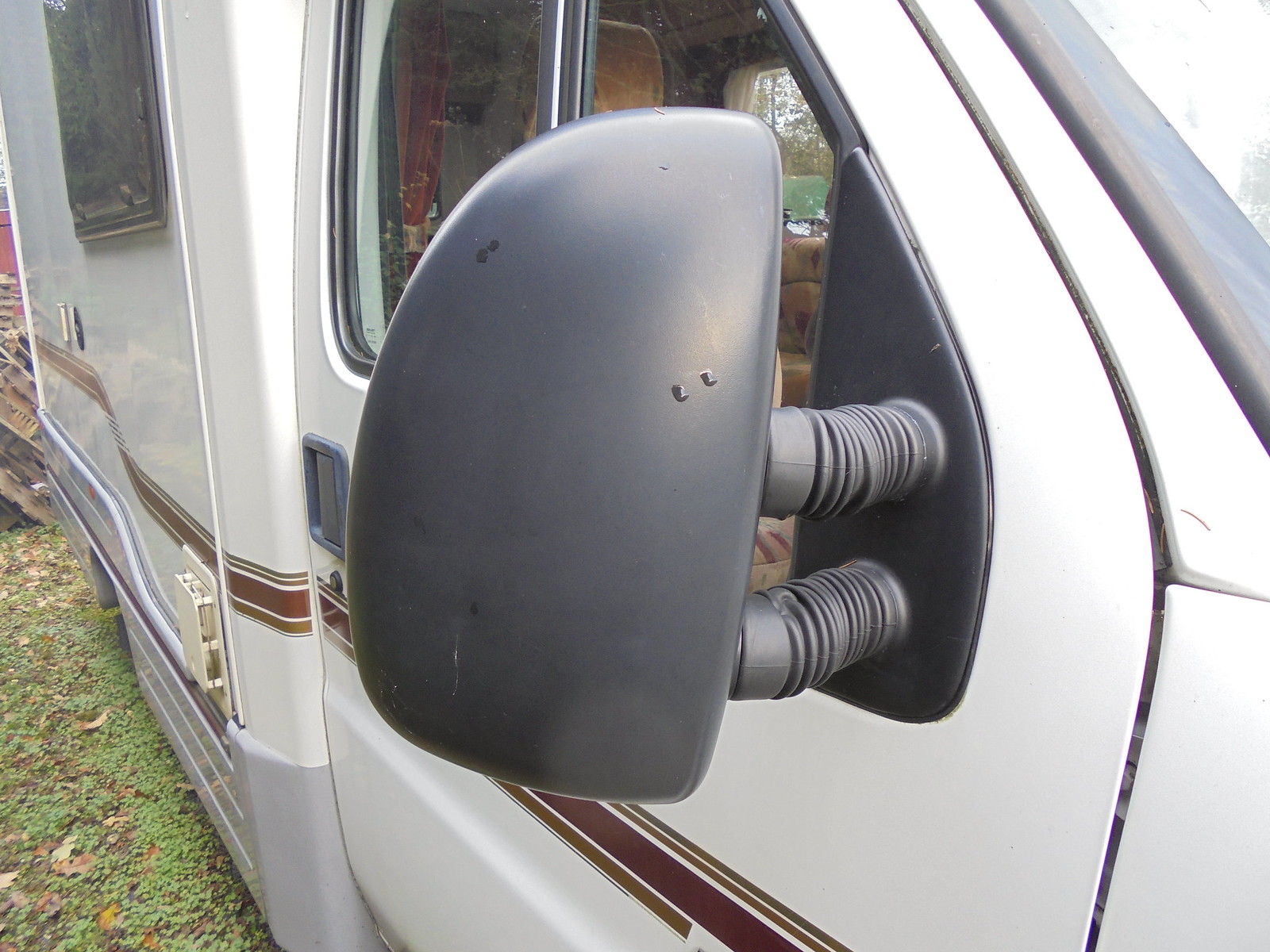This close-up photograph, taken outdoors on a cloudy day, features the right side of a white motorhome, heavily zoomed in on its rearview mirror. The mirror, encased in black plastic, is held in place by two gray collapsible rods, ensuring it is easily adjustable. This detailed view highlights the rearview mirror positioned against a large, clear window with a black lining. Along the white side of the vehicle, a dark brown stripe runs horizontally, accompanied by a couple of thin light brown lines above it, adding a touch of design. The vehicle, which is parked on grass, shows patches of green interspersed with tan areas at the bottom left of the image. The ground features a mix of green weeds and brown patches, suggesting a slightly worn or natural surface. Light enters from the top right corner, hinting at an open sky and lending a soft illumination to the scene.